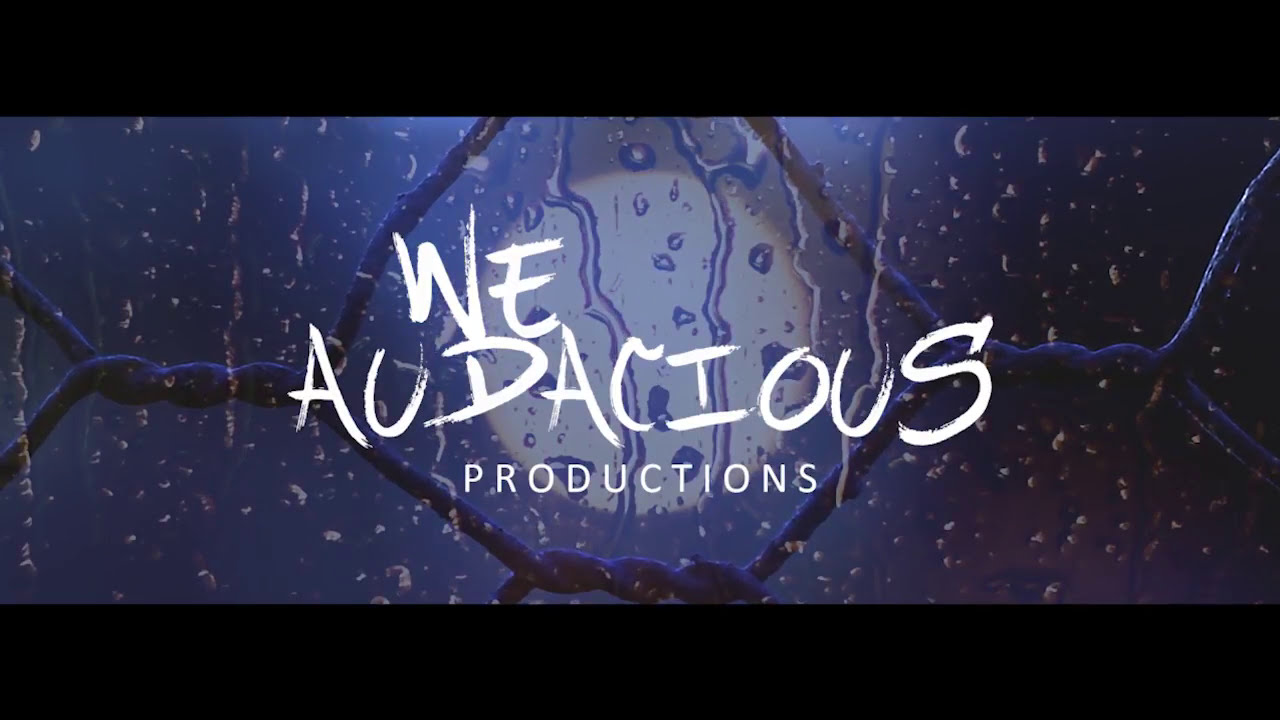The image features white text in the middle, reading "WE" on top and "AUDACIOUS" below in uneven, capitalized script, followed by “PRODUCTIONS” in a formal, evenly spaced font. These words are set against a close-up of a metal fence. Through a particular link in the fence, a round yellow light is visible, appearing to stare back at the viewer. Rain drips down the image, and the background is a bluish-purple night sky. The entire image has a letterbox format with black rectangles on the top and bottom, giving it a high-definition television shape—wider than it is tall.